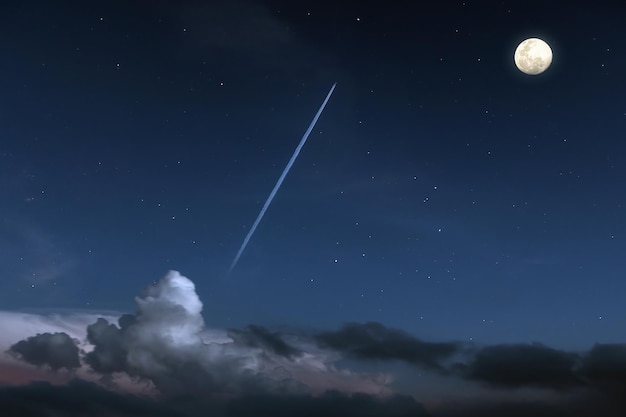In this animated image, a celestial scene unfolds under a dark blue night sky. At the bottom, dark gray clouds merge seamlessly with lighter purple and light gray variations, creating a gradient effect towards the center and left side of the image. Ascending above the cloud cover, the sky is punctuated by a luminous light blue shooting star, tracing a delicate arc across the scene. In the upper right corner, a vividly bright, circular moon casts its glow, dominating that quadrant. Scattered across the sky are numerous twinkling white specks, representing distant stars, adding depth and majesty to this serene nocturnal vista.